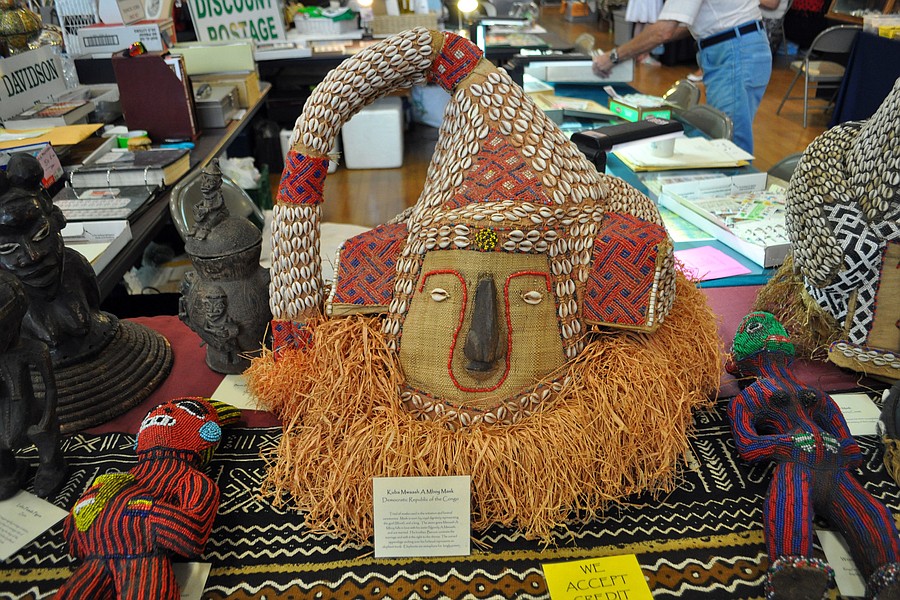The image is a full-color indoor photograph taken at what appears to be a craft fair or antique booth. The foreground features a table covered with a black blanket adorned with intricate white, gold, and brown tribal designs. Prominently displayed on the table is an aboriginal mask from the Congo, resembling an African Santa with a Santa-shaped hat decorated with puka shells, a coconut nose, and a light brown coconut grass beard. Various African artifacts are scattered around the table, including two dolls—one in red and blue striped clothes with a green head and another in black and red stripes with a red head. There's also a purse designed to look like a scarecrow amid the knick-knacks and books. A noticeable yellow post-it note on the table states, "We accept credit," hinting that the items are for sale. In the upper right corner of the image, an empty folding chair can be seen beside a man in blue jeans, a white short-sleeved shirt, and a belt, who is reaching for a box. Behind the main table are other tables cluttered with papers and possibly office equipment, along with people perusing the items.